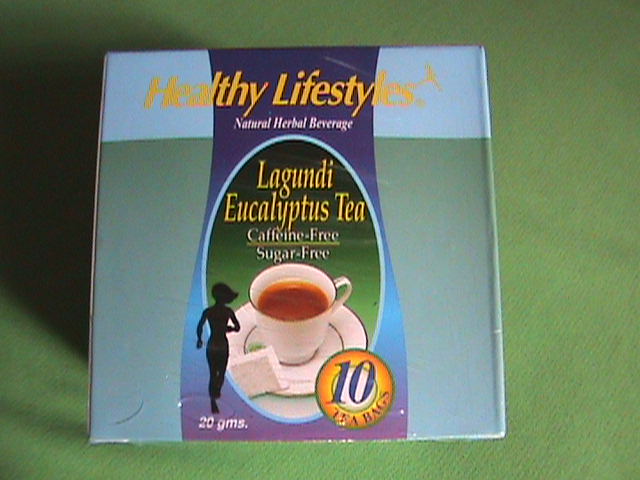The photograph captures a teabox set against a textured green fabric background with a prominent shadow cast towards the top left. The box has a light blue top section and a bluish-green bottom. Its center features a vertical purple strip taking up about one-third of the front, with a light blue oval in the middle that houses a green background with yellow lettering reading "Lagundi Eucalyptus Tea, Caffeine Free, Sugar Free." Below the oval is an illustration of a white teacup and saucer, with a sugar cube positioned at the 8 o'clock mark of the cup. To the left, there is a black silhouette of a running woman with "20 GMS" written beneath her. The bottom right corner has a yellow and orange circle with blue lettering indicating "10 tea bags." Above the purple strip, the yellow letters spell "Healthy Lifestyles," accompanied by the phrase "Natural Herbal Beverage."